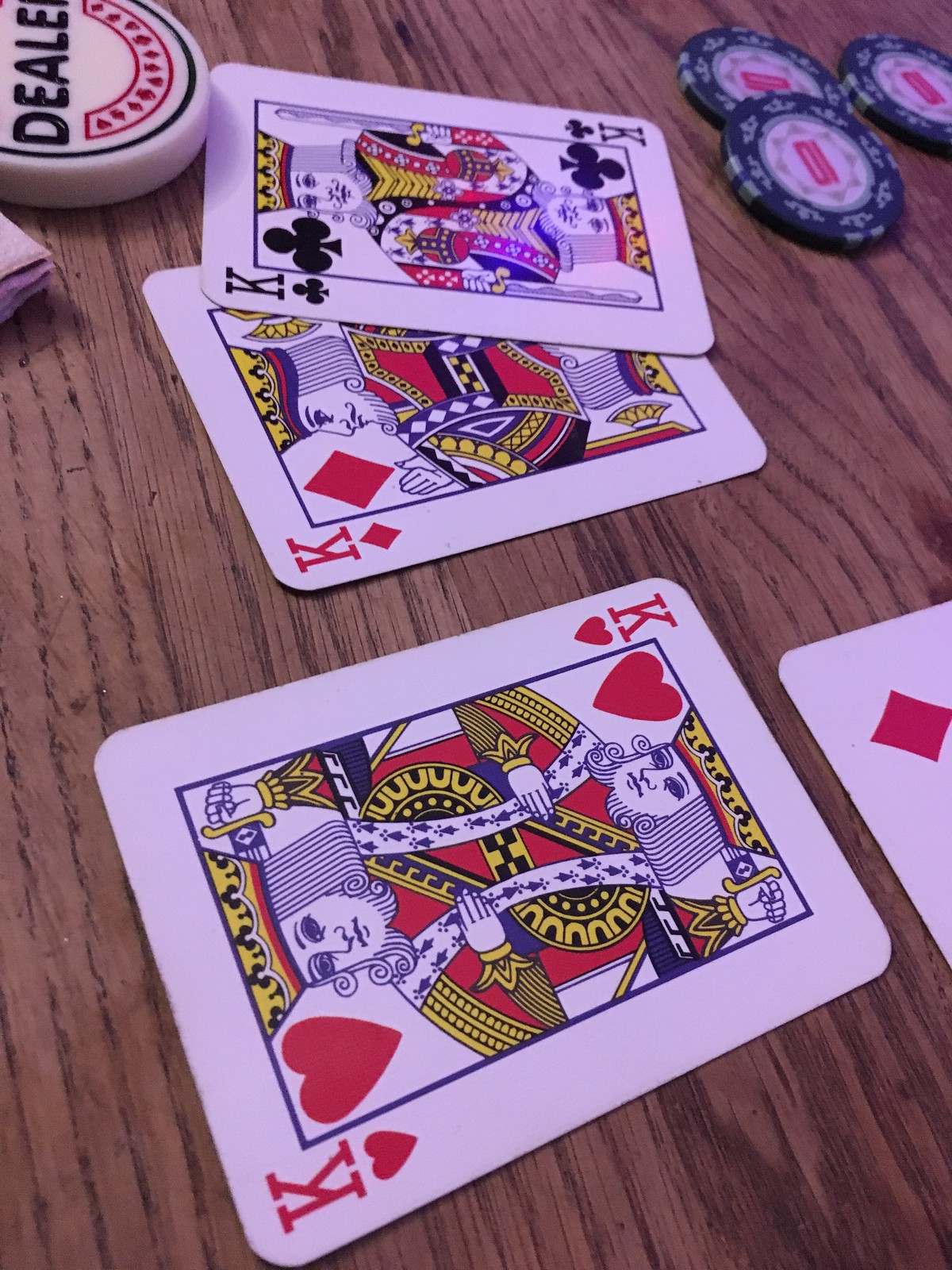This photograph features a medium to light brown wooden table with vertical grain patterns as the backdrop. In the upper left-hand corner, a round, off-white object labeled "dealer" in black letters is visible. Beneath it lies a red semicircle adorned with intricate designs. To the right of these items, two playing cards are positioned partially sideways, allowing the tops to be seen: a King of Clubs sits atop a King of Diamonds. In the upper right-hand corner, three blue poker chips are arranged, each featuring a blue rim, a white center, and a red square in the middle. Near the bottom of the image, a King of Hearts card is tilted slightly to the left, exposing its top left corner. In the center-right section of the photo, the corner of what appears to be another red card with a diamond symbol is also visible.